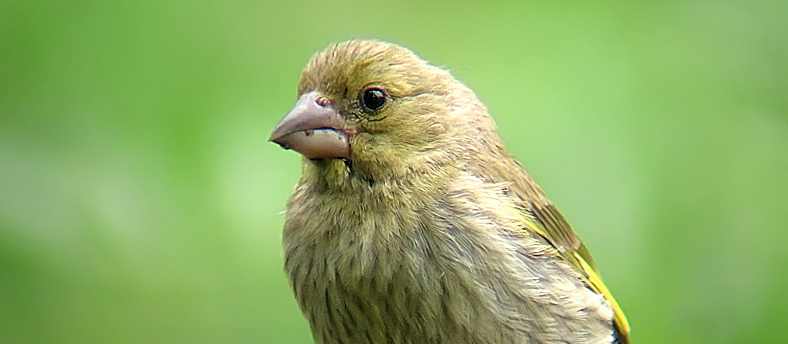The image showcases a close-up of a bird, beautifully captured with what seems to be a telephoto or macro lens. The bird is positioned centrally against a blurred green background, creating a soft, out-of-focus effect that highlights the bird's details. It has a rounded, fluffy head with light tan and white feathers, gradually transitioning into darker shades of tan towards the back, which resemble pin feathers. The bird's small, stubby, flesh-colored beak is pointed to the left and shows signs of some dirt or growths at the bottom. Its eyes are small, black, and encircled by lighter feathers, giving it a keen and attentive expression. The chest is adorned with fine white feathers interspersed with light yellow hues, while the wings exhibit more vibrant, bright yellow feathers mixed with brown. This detailed description emphasizes the intricate and delicate nature of the bird's plumage, creating a vivid image of its natural beauty.